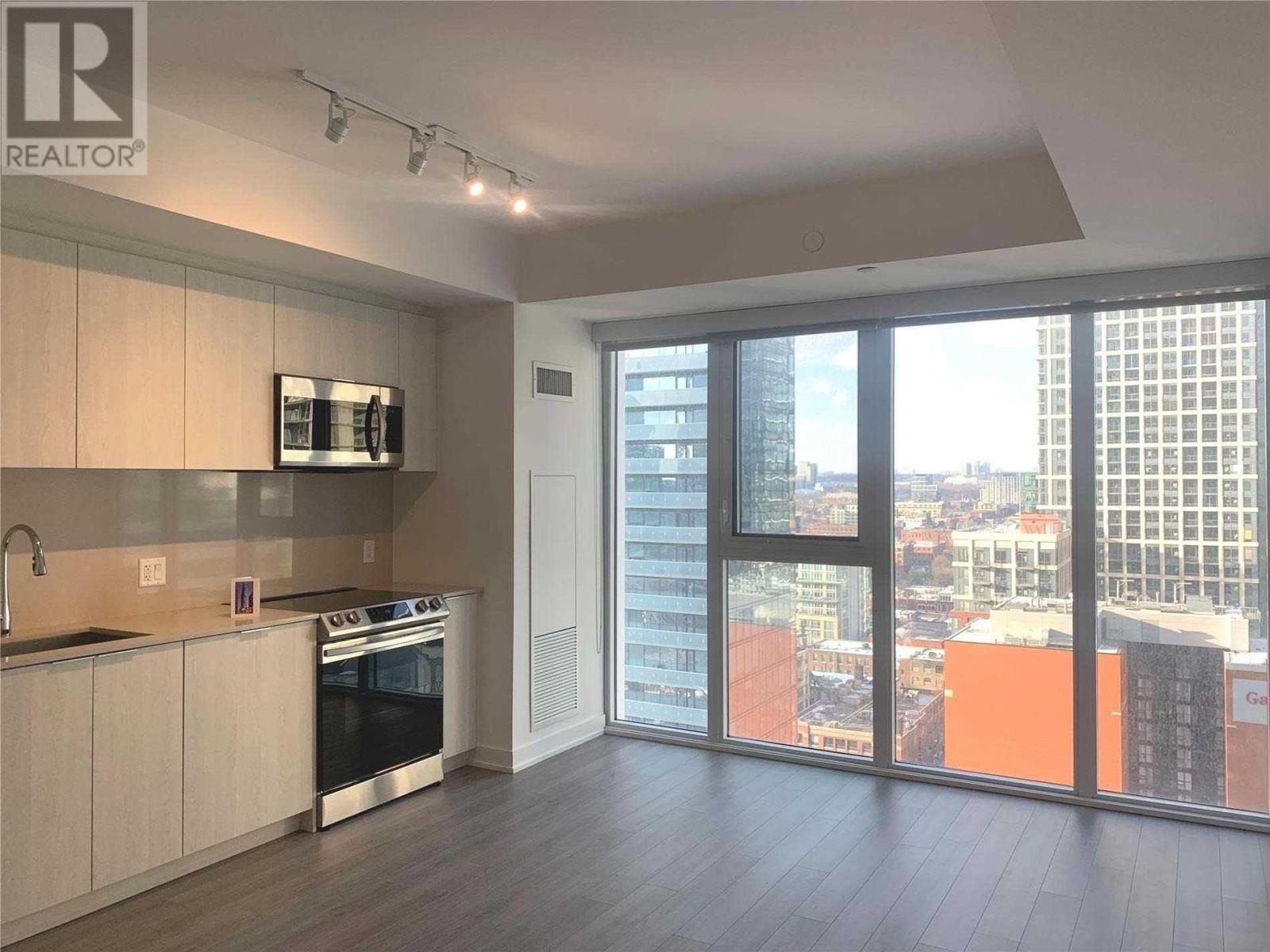A high-rise apartment interior is depicted in this photograph, showcasing two converging walls that meet at a corner. The dominant feature of the outer wall is an expansive window composed of five vertically-oriented sections. Four of the sections are tall, rectangular windows, with one of them split horizontally at the midpoint, possibly designed to open either inward or outward for safety. Beyond the glass, a cityscape filled with other tall buildings is visible.

The room features a floor with faux wood paneling and a white ceiling with a recessed area that houses track lighting. The interior walls are painted in a light gray hue, creating a cohesive and modern aesthetic. 

On the left side of the room lies the kitchen area, equipped with sleek, grayish-brown cabinetry. Above the stainless steel stove range is a microwave, and a sink is also present, seamlessly integrated into this stylish and functional space.